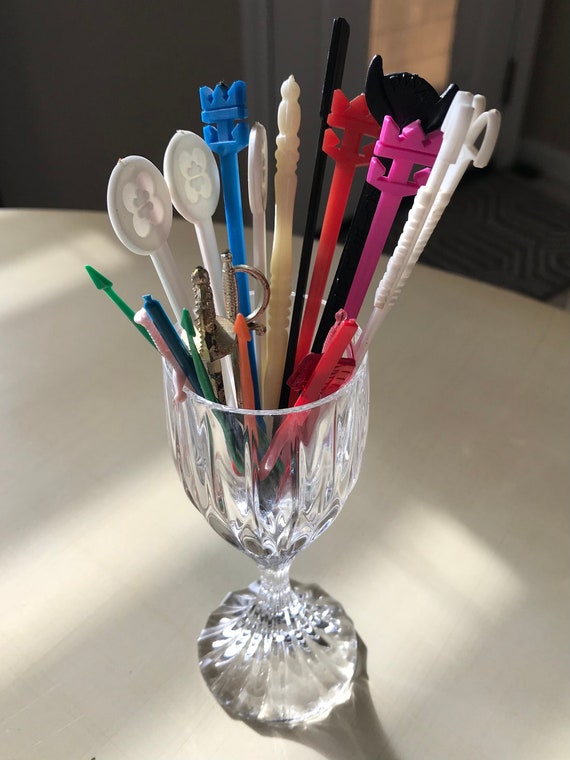The photograph showcases an intricately designed crystal-style wine glass, meticulously placed on a round table draped with a canvas-like white tablecloth. This elegant stemmed glass, set against the backdrop of a gray and red zigzag patterned carpet seen in the top right corner, is brimming with an eclectic assortment of decorative cocktail skewers. Among the skewers, vibrant colors such as pink, gold, black, red, blue, green, silver, and tan stand out. Each skewer is unique, featuring miniature swords, axes, and tridents, including a pink longsword, a gold-colored rapier, and a slim long black pick, while the smallest is a tiny gold sword. The detailed skewers, designed to resemble medieval weaponry and various fancy picks, contrast beautifully with the pristine white tablecloth and add a playful yet sophisticated touch to the setting. A nearby doorway with a window adds depth to the scene, making it a visually engaging composition.